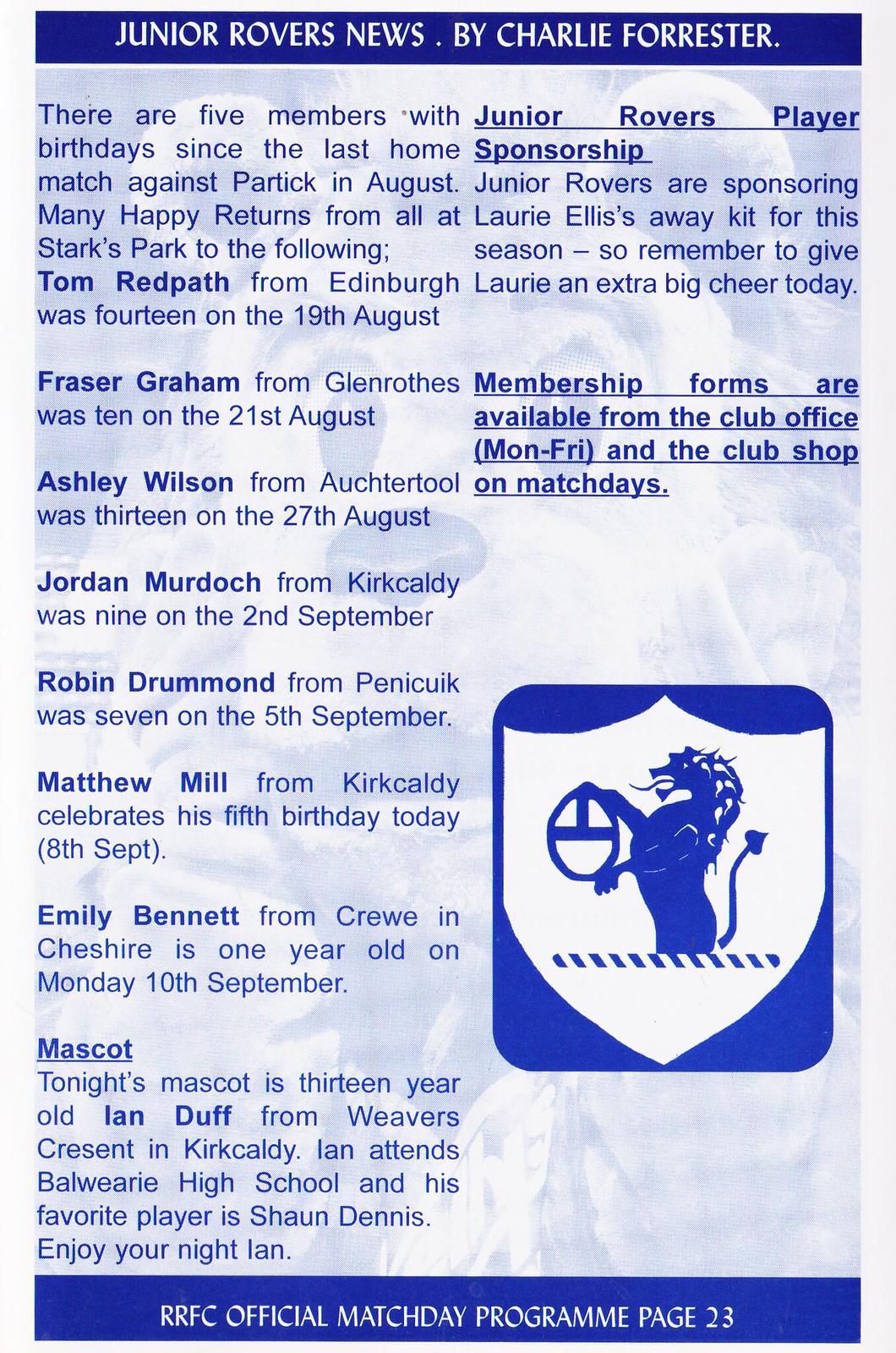This page from the "Junior Rover's News" by Charlie Forrester, featured in the RRFC Official Match Day Program on page 23, includes extensive text on a light blue background, accented with dark blue letters. At the top and bottom edges, blue rectangular borders encompass the titles and edition details. The top banner reads "Junior Rovers News by Charlie Forrester," while the bottom states "RRFC Official Match Day Program, page 23."

The faint background image appears to depict a sports mascot, likely a lion, rendered in blue, gray, and white tones. Overlaying this image, the text outlines various club member updates. Five members celebrated birthdays since the last home match against Partick in August, with well-wishes extended from all at Starks Park to Tom Redpath, Fraser Graham, Ashley Wilson, Jordan Murdock, Robin Drummond, Matthew Mill, and Emily Bennett, whose ages range from one to thirteen.

In addition, the page highlights specific details about the night's mascot, 13-year-old Ian Duff from Weavers Crescent in Kirkcaldy, who attends Ball Weary High School and favors player Sean Dennis. A section near the top right discusses Junior Rovers Player Sponsorship opportunities. Finally, a heraldic emblem is situated in the bottom right-hand corner, featuring a shield with a horse holding an egg and a pointy tail, emphasizing the club's identity.